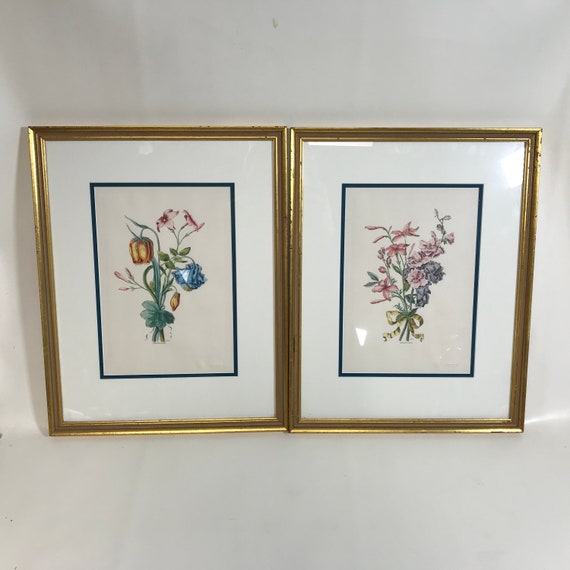This color photograph captures two framed botanical illustrations mounted side-by-side on a white wall. Each rectangular, glossy gold frame encloses a white mat featuring a narrow navy blue border at the edge. The illustrations themselves are set against a beige background. The one on the left showcases various flowers, including downward-hanging blue, orange, and pink blossoms, a red and yellow flower resembling a bell pepper, and yellow floral buds. Some of these flowers have stems with a bluish-green hue, adding to the intricate detail. The piece on the right displays more open-petaled flowers in shades of pink and purple, some of which are tied at the bottom with a yellow bow. The purple flowers resemble carnations, adding a textured variety to the meticulous floral arrangements.